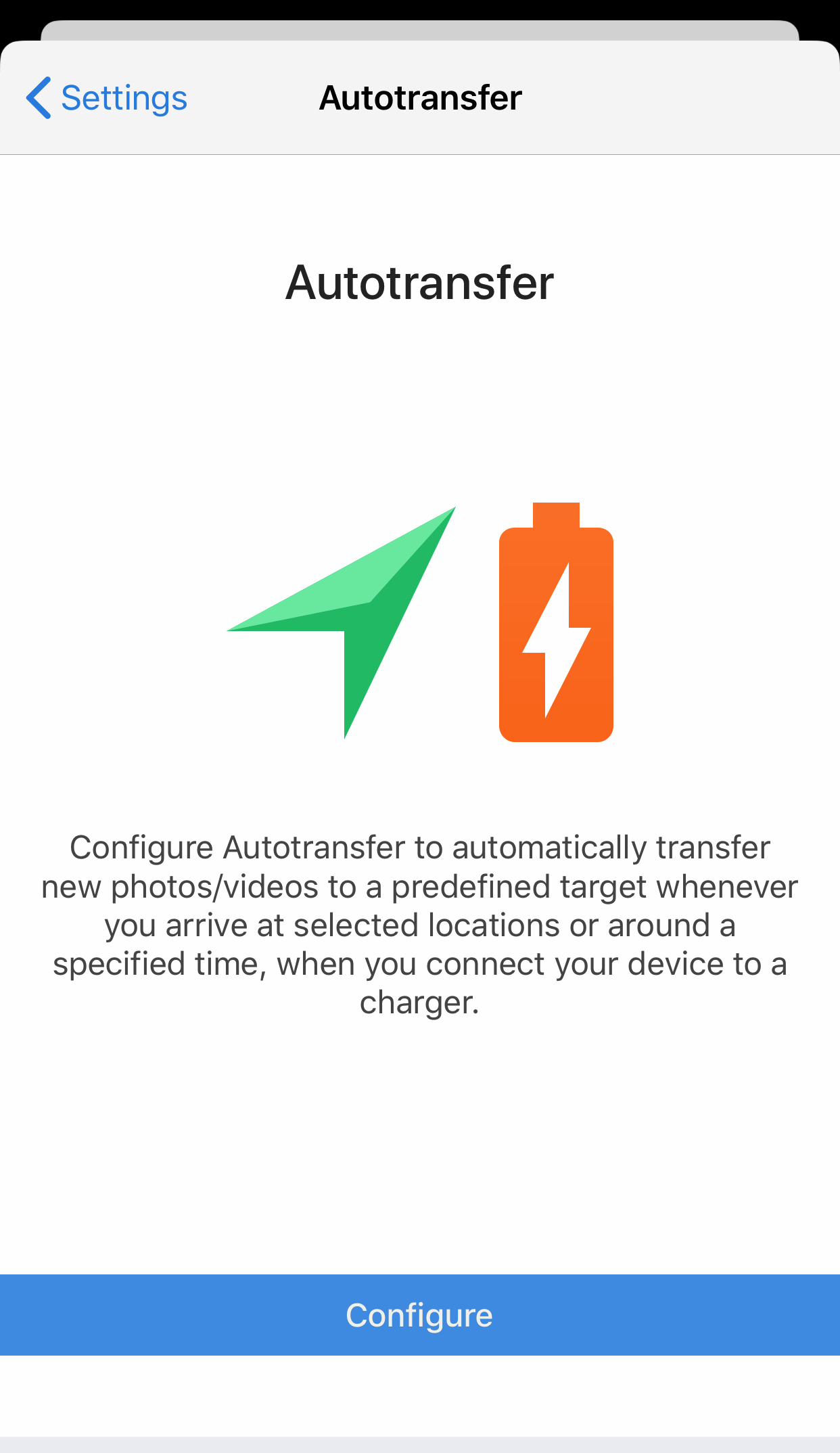The image features a white background with a thin black line at the top, followed by a slender light blue line just beneath it. Below these lines, there is a light blue box labeled "Settings," accompanied by a left-facing arrow and the text "Auto Transfer." 

Further down, on the white portion of the image, the words "Auto Transfer" appear prominently, accompanied by a green arrow pointing upwards and to the right. Adjacent to this is an orange battery icon with a white lightning bolt inside it. The text below the icons reads: "Configure Auto Transfer to automatically transfer your photos and videos to a predefined target whenever you arrive at selected locations or around a specified time when you connect your device to a charger."

At the bottom of the image, there's a blue box labeled "Configure," followed by a lengthy blue line stretching across the width of the image. The overall message conveys that the Auto Transfer feature allows for the automatic transfer of new photos and videos to a predefined target based on location arrival or specified times, particularly when the device is connected to a charger.